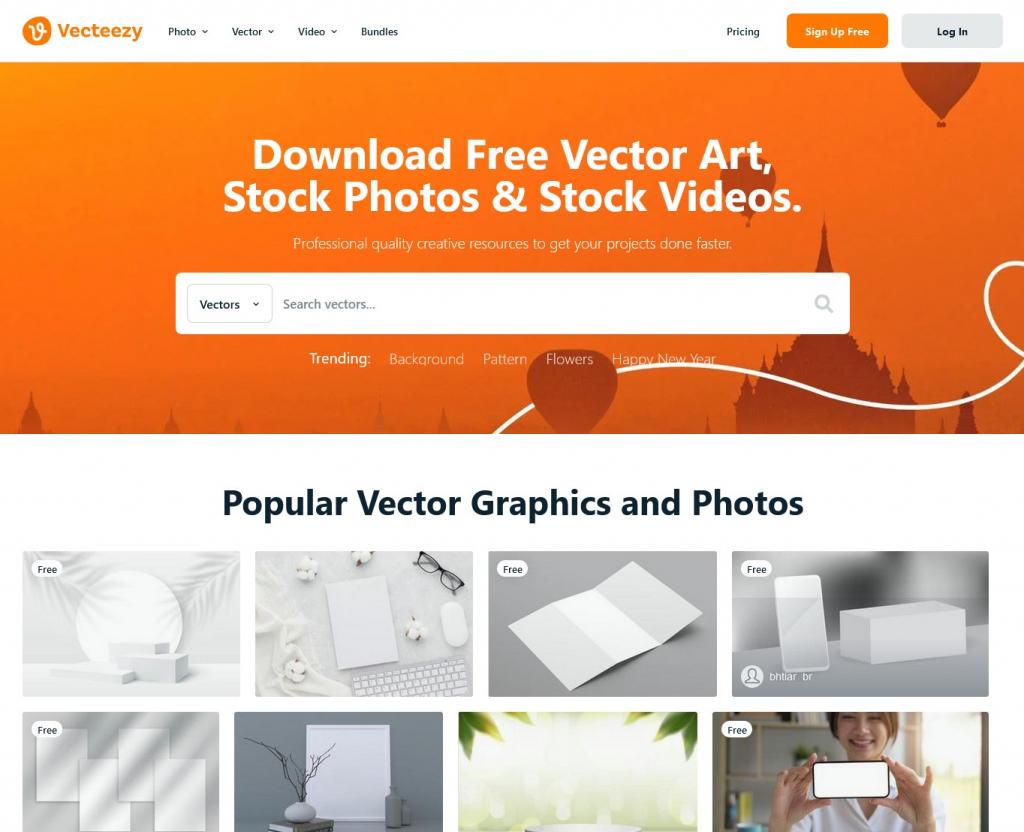The image is a screenshot from the website "Vecteezy." In the upper left-hand corner, there is an egg-shaped icon featuring a cursive letter 'V,' signifying the Vecteezy logo. Alongside the logo on the upper right, the website's navigation menu contains links to "Photos," "Vectors," "Videos," "Bundles," and "Blog," facilitating easy access to various types of content. The top right corner displays options for "Pricing," "Sign Up Free," and "Login."

Below the navigation bar, a prominent orangish banner features silhouettes of hot-air balloons, accompanied by the text "Download Free Vector Art." Underneath this banner, there are sections labeled "Stock Photos" and "Stock Videos," promoting Vecteezy's professionally curated, high-quality creative resources designed to help users complete their projects more efficiently.

Further down the page, there is a search bar specifically for vectors, indicated by a drop-down arrow next to the word "Vectors." Below the search bar, additional sections highlight "Popular Vector Graphics" and "Photos," offering users a curated selection of trending visual assets.